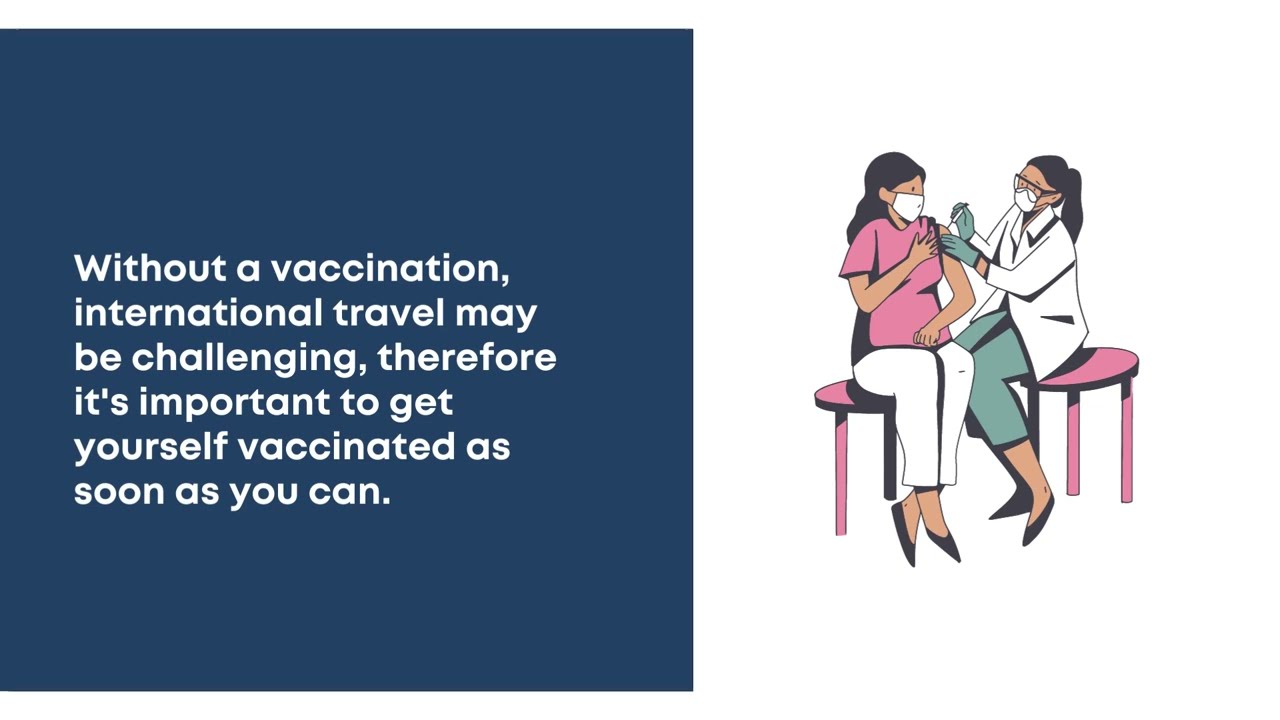The image is an informational medical banner promoting vaccination. On the left side, a blue box contains white text that reads, "Without a vaccination, international travel may be challenging; therefore, it's important to get yourself vaccinated as soon as you can." On the right side, there is a detailed illustration featuring a female medical professional and a patient. 

The professional, likely a doctor or nurse, has her hair tied back in a ponytail and is wearing a white lab coat, green pants, green gloves, black shoes, and a white face mask. She is holding a needle and administering a shot to another woman positioned to her left. The patient has her hair down and is dressed in a pink shirt with one sleeve rolled up to expose her shoulder, where she is receiving the injection. She also wears white pants and a face mask. Both characters are sitting on pink stools against a white background. The illustration is rendered in a simple, cartoon-like style.